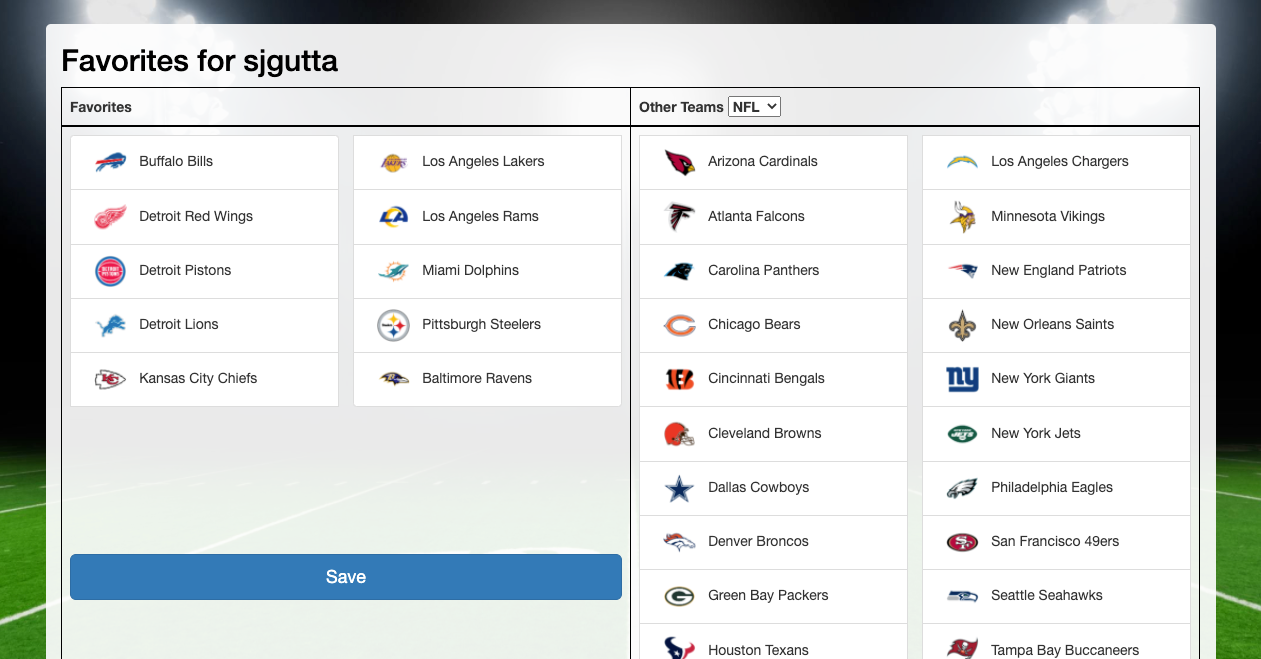The image displays a webpage showcasing a user's favorite selections among various NFL teams. The background features a football field along the bottom with a dark, black sky and stadium lights, but this is largely obscured by a prominent gray pop-up box dominating most of the page. 

In the upper left corner of the gray box, the title "Favorites for SJ Guta" is prominently displayed. Below this title, there is a structured table divided into two primary sections. Each section contains two sub-columns presenting the favorite teams.

The left section, titled "Favorites," lists ten sports teams, each accompanied by their respective logos situated within white rectangular boxes and separated by gray dividing lines. The teams are as follows:
- Buffalo Bills
- Detroit Red Wings
- Detroit Pistons
- Detroit Lions
- Kansas City Chiefs

The right sub-column under "Favorites" includes:
- Los Angeles Lakers
- Los Angeles Rams
- Miami Dolphins
- Pittsburgh Steelers
- Baltimore Ravens

At the bottom of the "Favorites" section, there is a prominently displayed Save button with a blue background and white text reading "Save." This button extends the full width of the section and is the same height as each individual row.

The other major section of the table consists of a drop-down menu labeled "NFL," indicating the remaining NFL teams alphabetically arranged in two columns. The first column spans from the Arizona Cardinals to the Houston Texans. The second column continues from the Los Angeles Chargers to the Tampa Bay Buccaneers, maintaining alphabetical order.

Overall, the detailed layout effectively highlights the user's preferred teams and provides an intuitive interface for managing these selections.